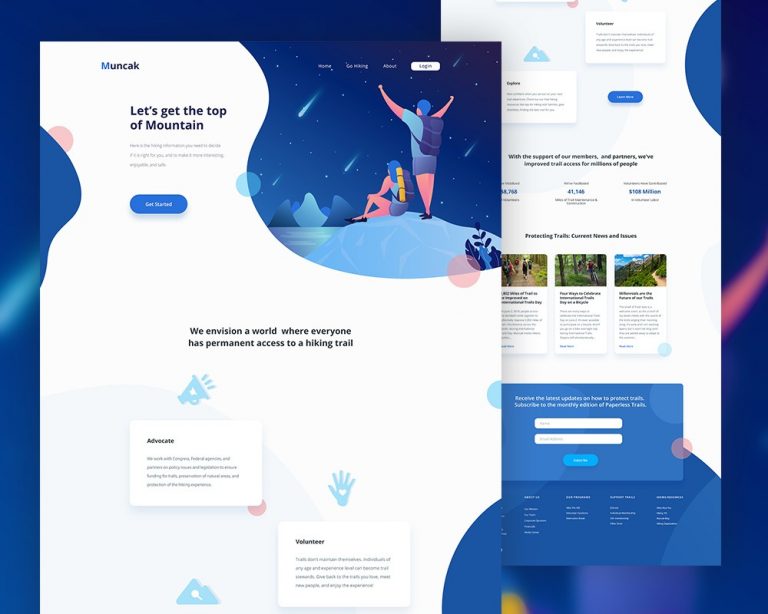The image features a predominantly bluish border background with hints of other colors subtly integrated. It includes various pop-up windows positioned across the scene. On the upper left, a distinctive white overlay displays the word "Mooncock" in dark blue text, accompanied by the slogan "Let's get to the mountain or the top of the mountain" and some fine print that is not legible. Beneath this text, a blue oblong button with the phrase "Get Started" stands out.

The remainder of the image is mainly white or off-white, dotted with several pop-up windows bearing titles like "Adventure" and "Volunteer," although the print beneath these titles is faint. Various icons, including a tooting horn, an outstretched hand, and a mountain, are scattered within this section.

Towards the top, there is a small, white menu with hard-to-read text. The central visual depicts a man standing triumphantly on a mountain peak with his arms outstretched and a backpack on his back, alongside a woman seated before him. They appear to be gazing at a cascading meteor shower set against a night sky. A small bush is visible at the bottom of this scene.

To the right, a rectangular pop-up window is prominently displayed, adding to the intricate composition of the design.